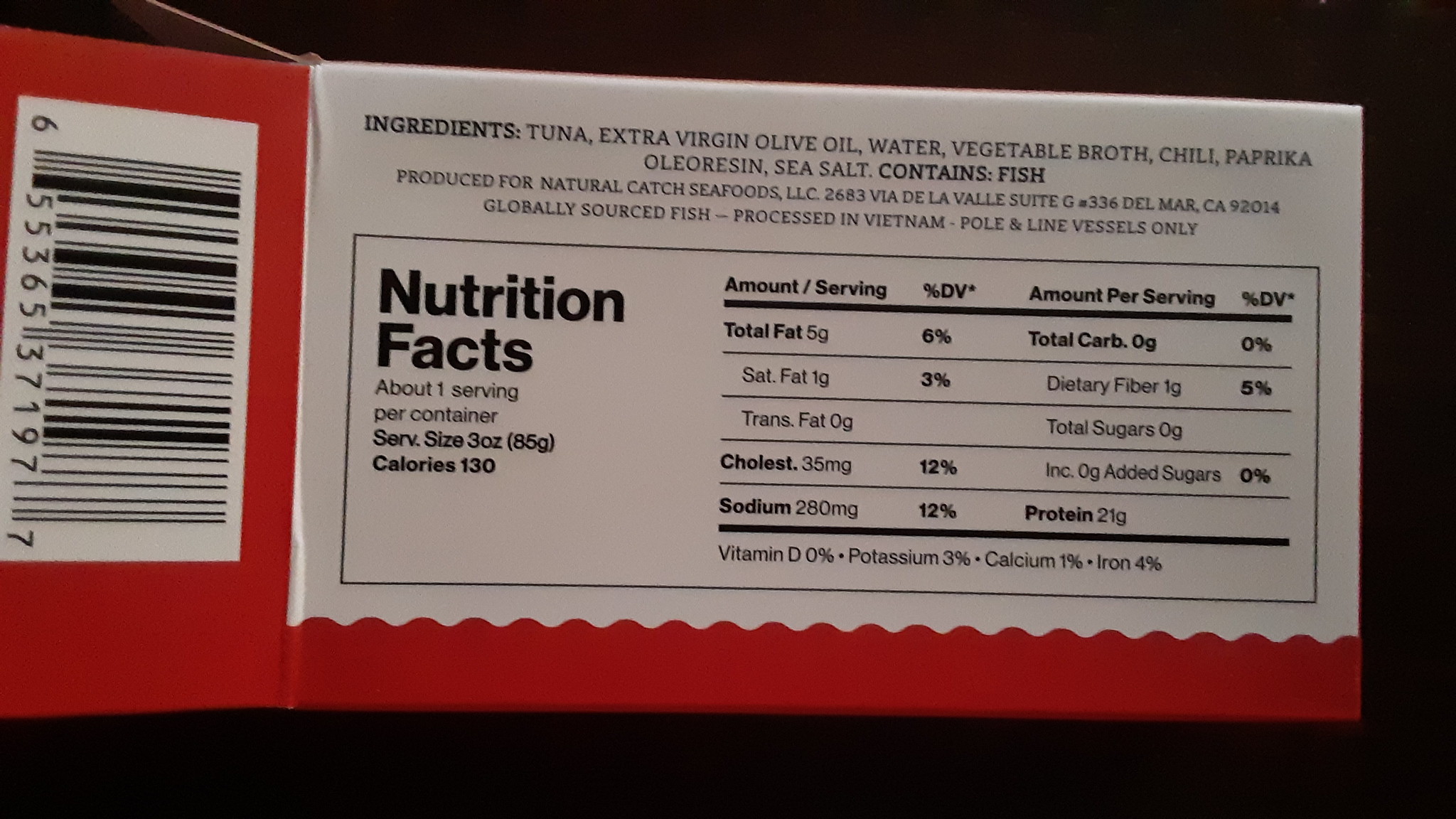The image depicts a small, predominantly red retail tuna box, positioned sideways against a black background. The left flap of the open box features a barcode. The center highlights a white label with black text detailing both the ingredients and the nutrition facts. The ingredients list includes tuna, extra virgin olive oil, water, vegetable broth, chili, paprika, oleoresin, and sea salt, and it notes that the product contains fish. It emphasizes that this tuna is produced for Natural Catch Seafoods, LLC, with an address in Del Mar, California. The fish is globally sourced and processed in Vietnam, using pole and line vessels only. The nutrition facts label outlines that the package contains one serving per container weighing three ounces, delivering 130 calories. Key nutritional values include 6% fat, 3% saturated fat, 12% cholesterol, and 12% sodium.